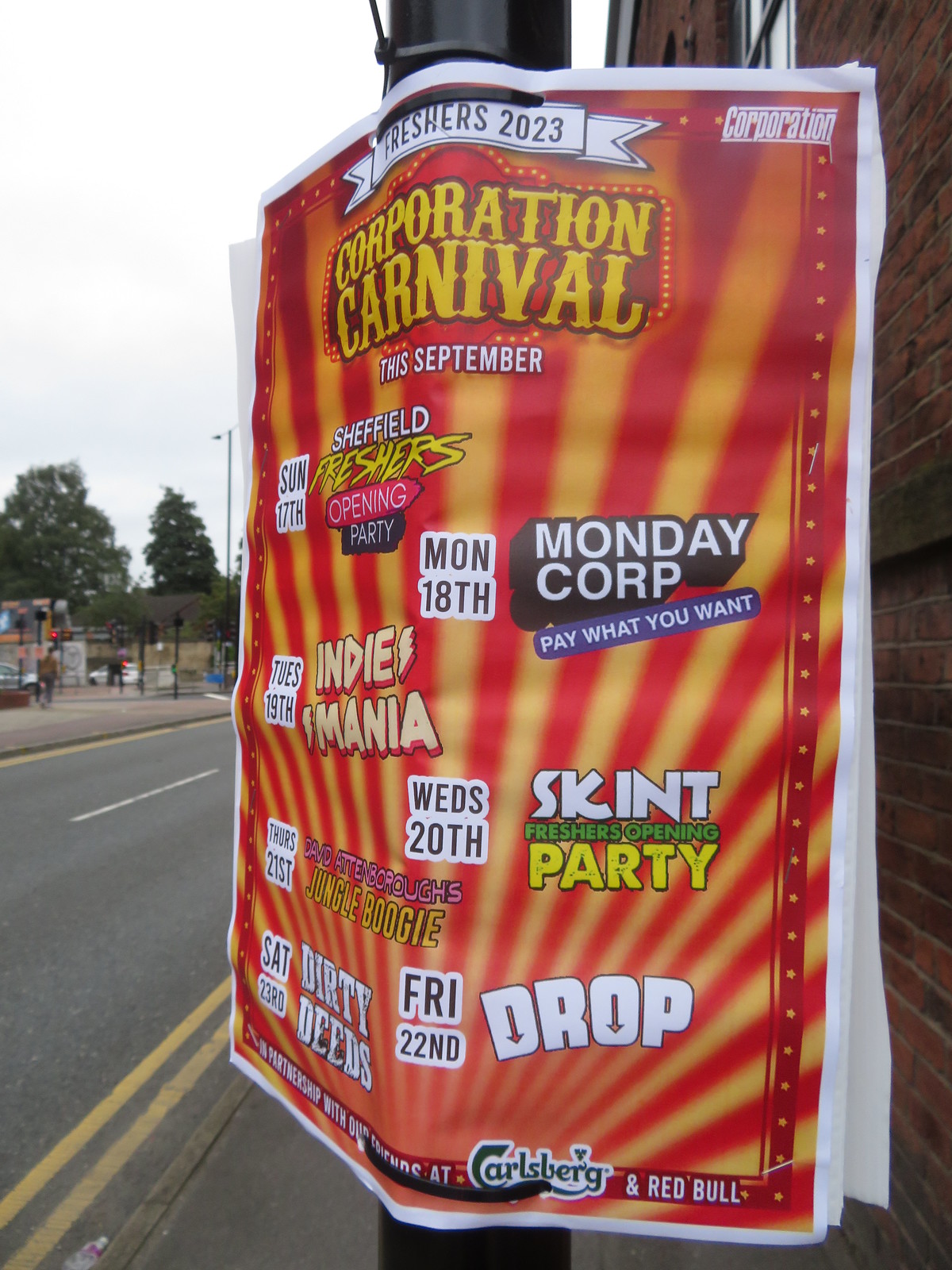The image showcases a detailed flyer taped to a black pole on the side of a street. The flyer features an eye-catching background that transitions from yellow to orange, resembling rays of the sun spreading outwards. It prominently displays a white banner at the top with the text "Freshers 2023," accompanied by "Corporation" in white letters to the right. Below, in yellow letters against the orange background, it reads "Corporation Carnival." Further down, in white text, it announces the event is taking place "this September."

A schedule of events is listed as follows:
- "Sunday the 17th: Sheffield Freshers Opening Party"
- "Monday the 18th: Monday Corp (Pay What You Want)"
- "Tuesday the 19th: Indie Mania"
- "Wednesday the 20th: Skint Freshers Opening Party"
- "Thursday the 21st: Jungle Boogie"
- "Friday the 22nd: Drop"
- "Saturday the 23rd: Dirty Deeds"

In the bottom right corner, the logos for Carlsberg and Red Bull are visible. The flyer is mounted on a black post; to the right side, a red brick wall is visible, and to the left, an asphalt street with double yellow lines and a central white line can be seen. Across the street, there are trees, an electric pole, and a gray-walled building with several people walking by. Additionally, a bottle of water with a purple label lies on the street in the bottom left corner.